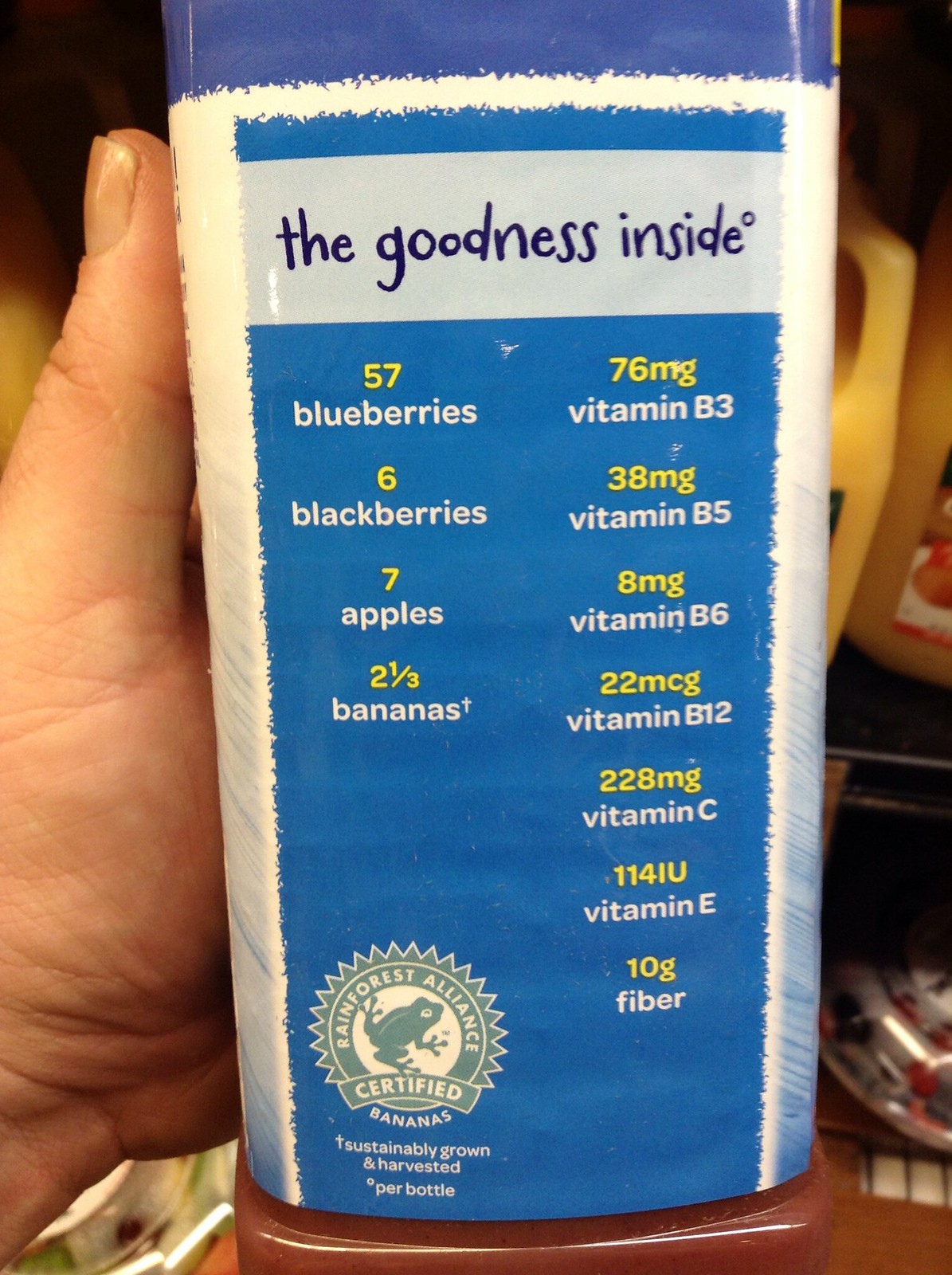In this close-up image, a Caucasian hand is holding a bottle with a blue wrapper. The actual bottle appears to be brown, which is partially visible at the base where the plastic part can be seen. The wrapper prominently features the text "The Goodness Inside" within a large blue rectangle. Detailed nutritional information is also listed on the wrapper, including the presence of 57 blueberries, 76 milligrams of vitamin B3, 6 blackberries, 38 milligrams of vitamin B5, 7 apples, 8 milligrams of vitamin B6, 2 1/3 bananas, and 22 micrograms of vitamin B12, among other ingredients. Additionally, the wrapper displays the Rainforest Alliance Certified symbol with a tree frog on the bottom left, indicating sustainable sourcing.